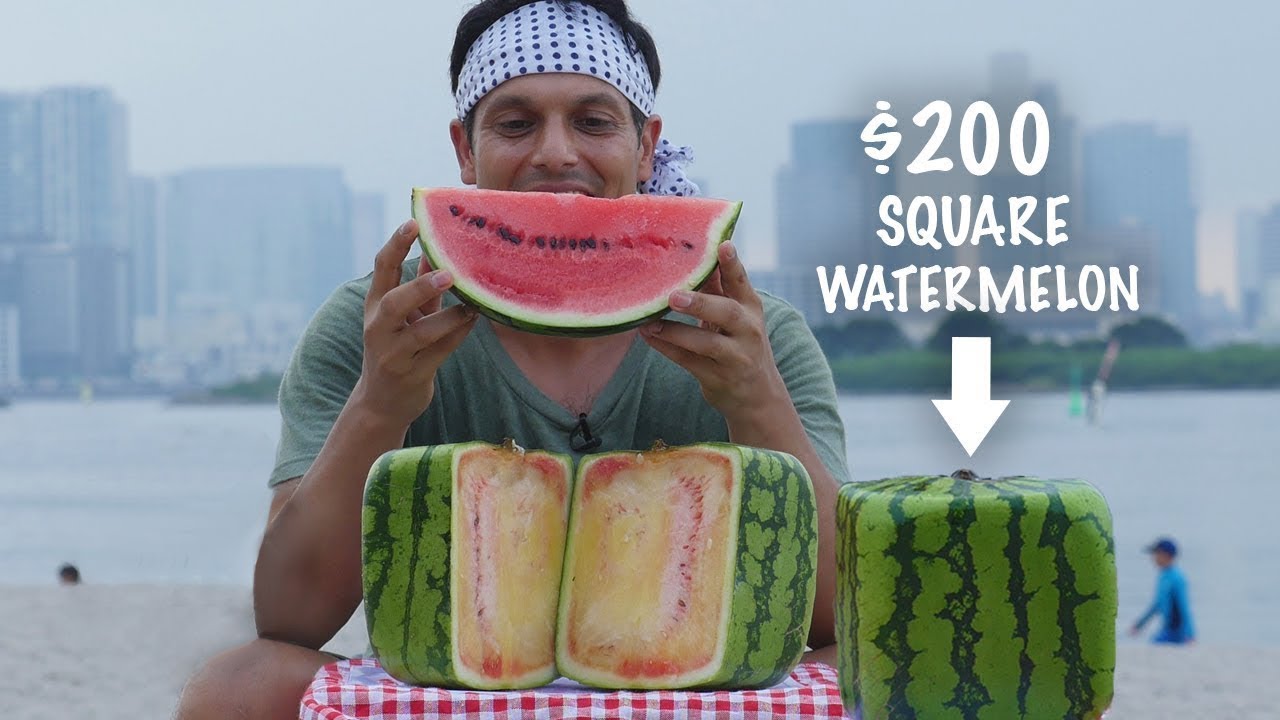In this photograph, a man at a beachside setting is about to enjoy a piece of watermelon. He is centrally positioned at a table adorned with a red and white checkered tablecloth. The man sports a green V-neck shirt and a white headband with black dots. Holding up to his face is a large slice of watermelon with a vibrant red interior and black seeds, positioned like a smile.

In front of him on the table, a distinctive square watermelon is prominently displayed, accompanied by a sign that reads "$200 square watermelon" with a white arrow pointing downwards. Another square watermelon is shown cut open next to the sign on the table. The background reveals a large body of water, possibly a lake or ocean, with pedestrians moving along the shore. Further back, a cityscape with buildings is visible, contributing to the bustling beachfront ambiance. The image captures the man’s focus on enjoying his watermelon, juxtaposed with the intrigue of the costly and uniquely shaped square watermelon.